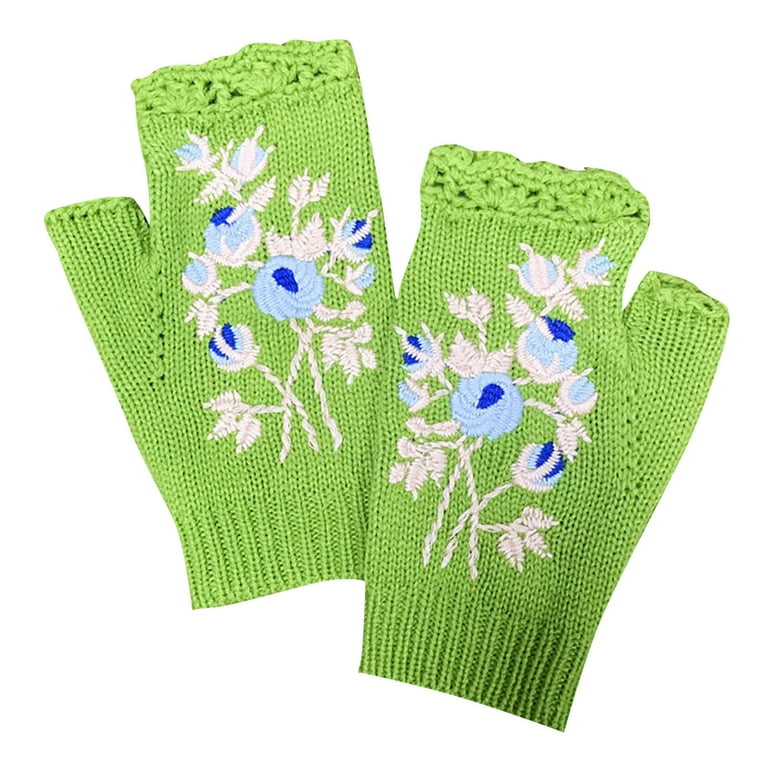This image features a pair of bright green, knitted fingerless gloves set against a completely white background. The left glove, with its thumb facing outward, is positioned on the left side of the image, while the right glove is on the right side. The gloves are ribbed at the wrist for a snug fit and have a crocheted section where the fingers go, giving them a delicate lace-like appearance. The thumb holes are stitched around the edges and are located on the outer sides of each glove. The top of each glove is adorned with an intricate embroidery of white stems and leaves, topped with light blue blooms that have dark blue centers, providing a charming decorative touch.